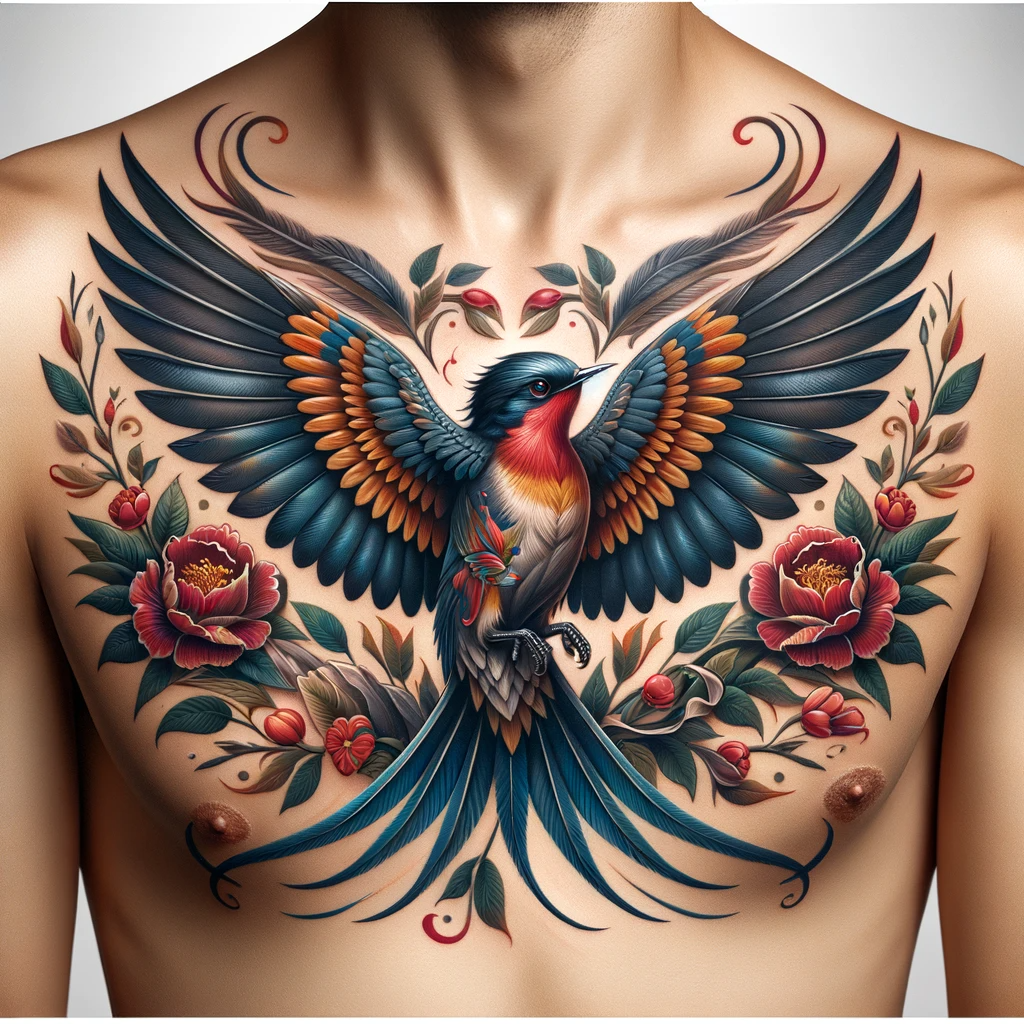This image appears to be an AI-generated depiction of a man's upper torso, predominantly featuring an intricate tattoo. The main element of the tattoo is a vibrant bird, positioned centrally on his chest. The bird displays an array of colors; its head is adorned with blue feathers, transitioning to red along its breast, then to orange, and ultimately back to blue for its tail. The wings, extending to the left and right, showcase an elaborate design with blue and orangish-yellow hues, eventually transforming into various shades of blue towards the edges. Below the bird and spreading around its base are several wreaths of red roses, which also have green leaves interspersed among them. Some of these leaves appear to have small berries growing from them. The overall image is characterized by a shiny, computer-generated appearance, emphasizing the detailed and colorful nature of the tattoo.